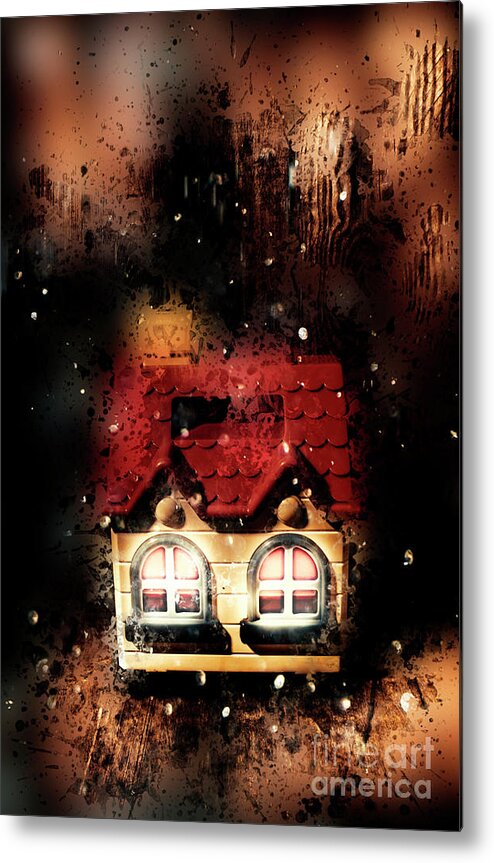The image showcases a digital, highly dramatic artwork resembling a blend of photography and painting, prominently branded with "Fine Art America" in the bottom right in thin, light grayish-white text. The scene depicts a small, quaint cottage, with a distinct red roof and two bright, light-filled windows, suggesting a cozy, one-room living space. The artwork features inconsistent shadows and a black background, creating a mysterious atmosphere reminiscent of a horror scene. The background includes orange lights and is speckled with raindrop effects, adding to its surreal, dream-like quality. The entire piece has a splattered, spray-painted look with bright gold, green, and bronze colors, and it exhibits a texture suggesting both digital and physical media, rounded off with abstract elements that give it a unique, tactile feel.